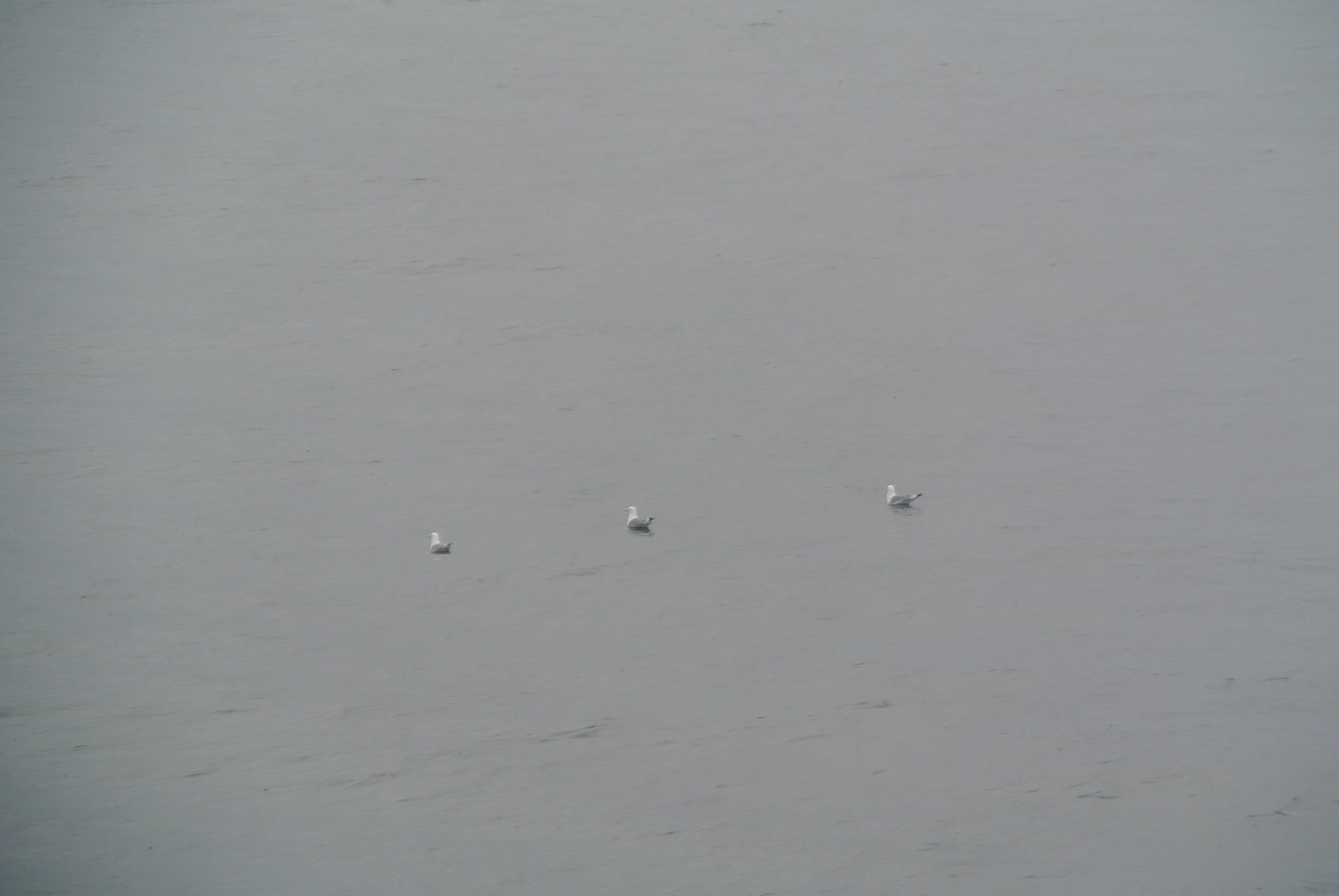The image depicts a serene, nearly monochromatic scene of a calm body of water, possibly an ocean or lake, with a predominantly gray hue, offering little to no blue tones. The water surface is almost entirely still, exhibiting only a few slight ripples near the bottom of the frame. Dominating the center of the image are three birds with white heads, gray feathering on their backs, and black-tipped tails. These birds are aligned in a straight formation across the water, giving them a synchronized appearance. The bottom left corner of the image is slightly darker, suggesting a shadow or a focus effect, but adding no significant additional elements. The minimalist and uniform layout, with its muted colors and repetitive pattern, emphasizes the tranquil nature of the scene.